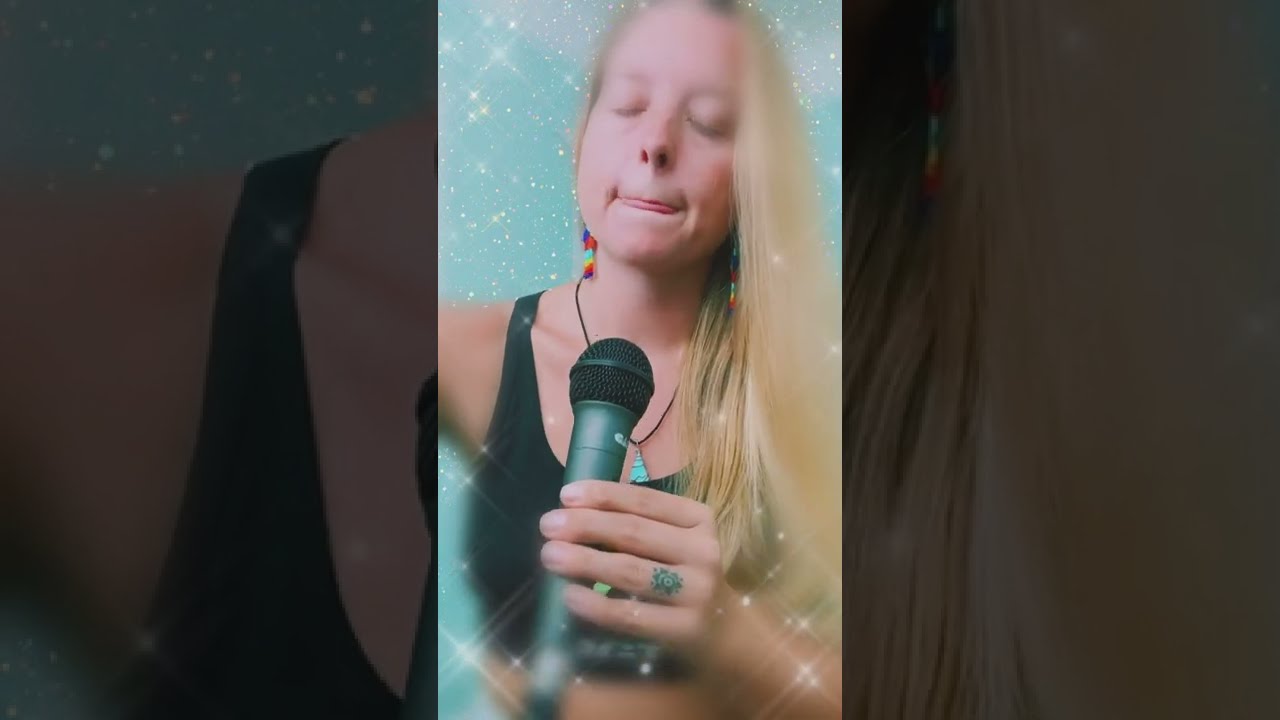In the center of the image stands a young woman with long, blonde hair cascading past her shoulders. Her eyes are closed and her lips are pursed, with a small part of her tongue visible. She wears a black sports bra and holds a black microphone with her left hand, barely grasping it. Prominently, she wears a black string necklace adorned with a turquoise triangle pendant. Her left ring finger sports a green ring, and one of her hands showcases a tattoo. Long, colorful earrings featuring shades of red, teal, yellow, and purple dangle from her ears. The background is a vivid green, adorned with numerous white, sparkling lights that create a glittery overlay both behind and in front of her, adding a surreal, magical quality to the scene.